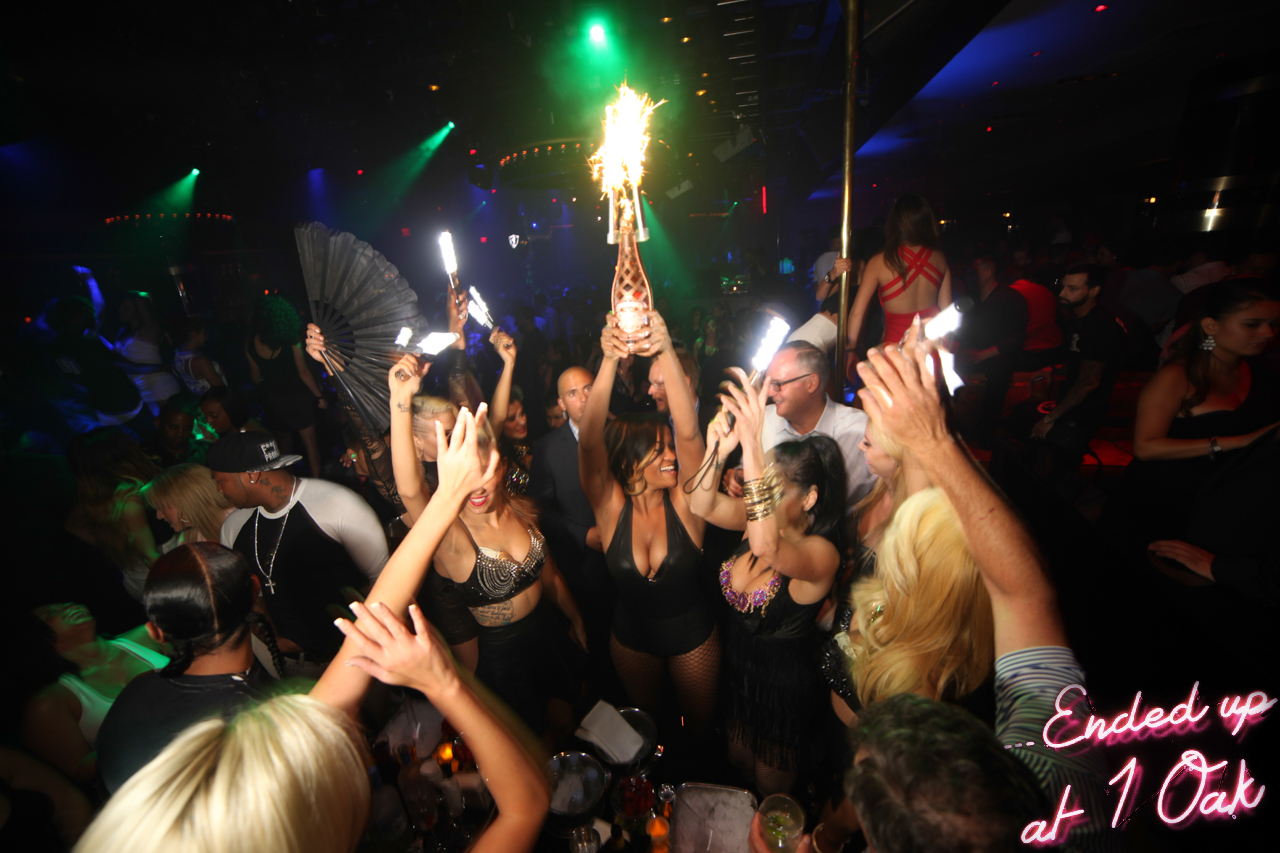The photograph captures a vibrant and crowded party scene inside the One Oak club. The foreground is dominated by a group of smiling women enthusiastically raising a bottle of liquor and brightly lit objects, contributing to the festive atmosphere. Surrounding them are a mix of men and women, all engaged in the lively celebration. The background reveals a dazzling array of strobe and neon lights in green, blue, and red hues, casting an energetic and colorful glow over the packed dance floor. The density of the crowd, dressed in trendy night-out attire including some swimsuits, underscores the club's bustling and spirited nightlife. The lower right corner of the image features stylized white cursive text that reads "ended up at One Oak," signifying the popular club where this exuberant gathering is taking place. Overall, the scene exudes a sense of enjoyment and revelry, epitomizing the dynamic party ambiance that One Oak is known for.